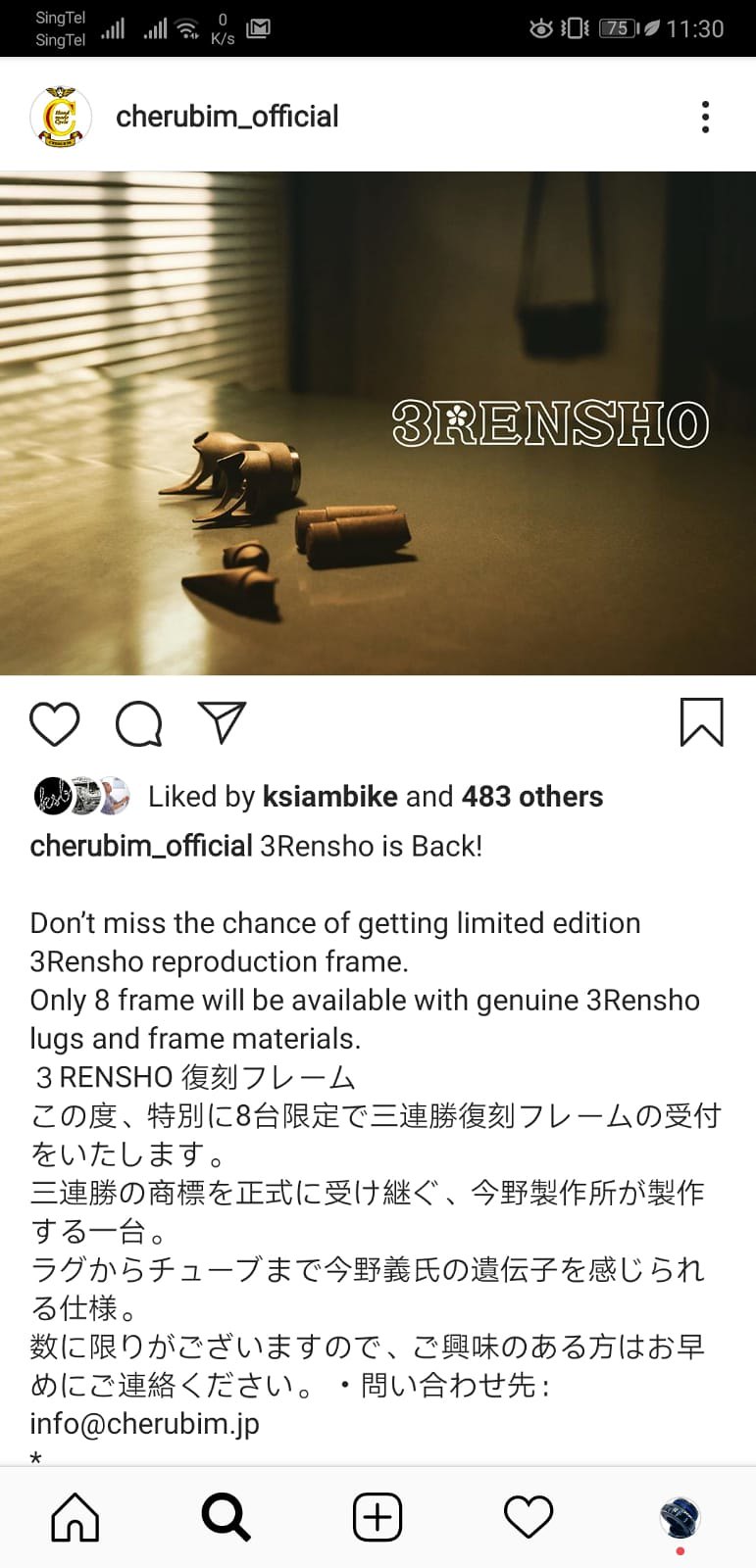The screenshot, taken on a mobile phone at 11:30 with 75% battery, captures an Instagram post from the account @cherubim_official, which prominently displays the announcement: "3RENSHO is back! Don't miss the chance of getting a limited edition 3RENSHO reproduction frame. Only 8 frames will be available with genuine 3RENSHO lugs and frame materials." The image shows a table with what appears to be destroyed pen-like objects or wood shavings, situated in front of a window with closed blinds. A blurry bag or purse hangs on the wall in the background. The screen also features various symbols, including Wi-Fi logos, and Asian writing below the promotional text. The post has been liked by KSIAMBike and 483 others.